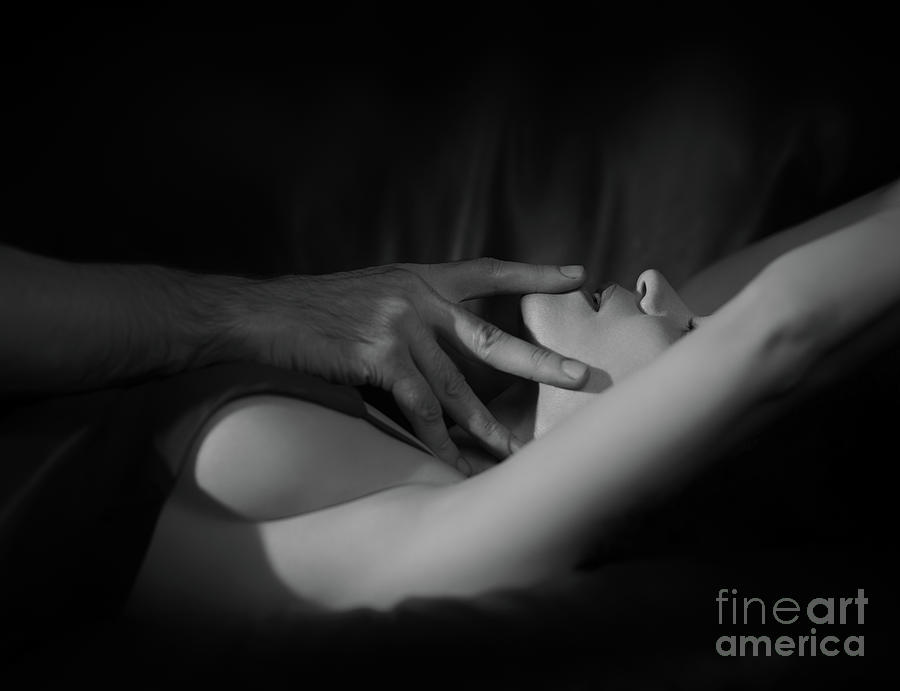In this black and white erotic photograph, a woman with lighter skin is lying on her back on a dark, comfortable surface, with her head resting on a pillow. Her arms are stretched behind her head, accentuating a revealing pose, while she wears a silky, dark nightie or negligee that exposes significant sideboob. The background features a dark, silky sheet hanging down, adding to the sensual ambiance. From the left side of the image, a man’s hairy arm appears, reaching over her breast area and sensuously touching her chin and the bottom of her lip with his fingers. This image, with its focus on the woman’s exposed figure and the man’s intimate gesture, captures a highly provocative and sensual moment. In the bottom right corner, a light gray watermark reads "Fine Art America."